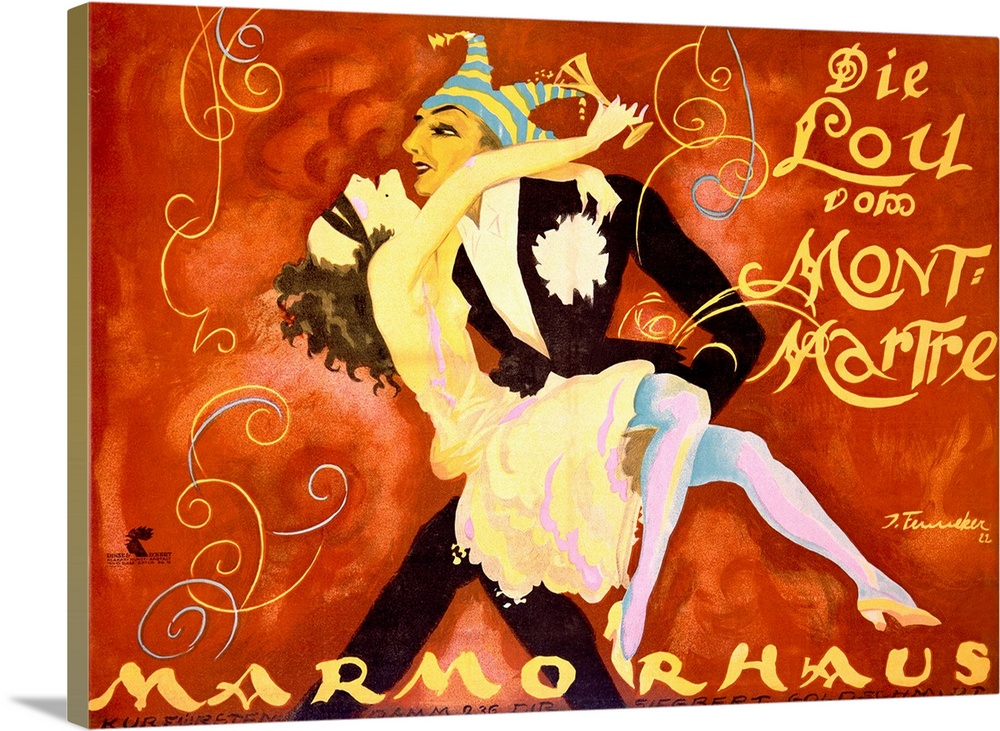The image depicts a dramatic canvas print styled like a book cover from the 1920s and 30s, characterized by vibrant and expressive details. At the center is a man wearing a black suit adorned with a white boutonniere, a blue and yellow jester hat, and makeup featuring red lipstick. The man has his arms around a woman who is wearing a thin, pale yellow dress and yellow high heels. She has curly brown hair, her head tilted back, and appears to be holding a tilted wine glass with its contents spilling slightly. The background is a burnt auburn color, accentuating the bold yellow font of the title "D. Lou Dommement Marcher." At the bottom, the artist or author’s name "Marmo Rouse" is displayed alongside the word "Marmocos." The image evokes a sense of theatrical drama, possibly suggesting a dance or embrace, with the man's hand intriguingly placed underneath the woman's dress. The overall style and elements bring forth an atmospheric and enigmatic aura, typical of early 20th-century poster art.